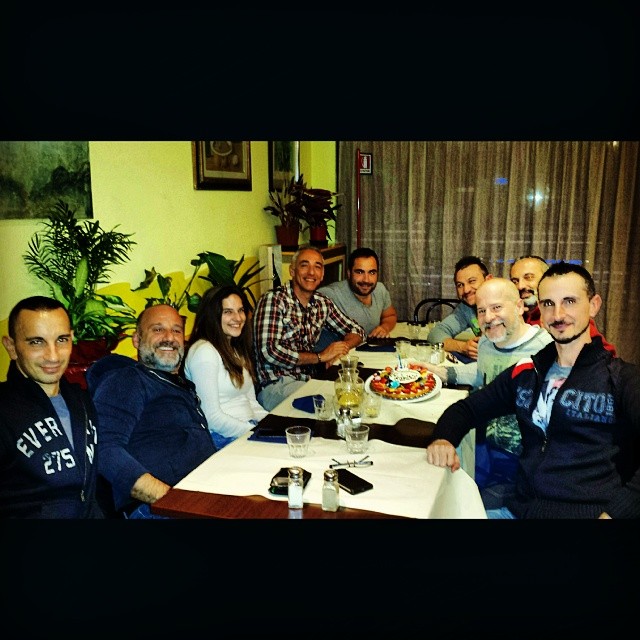In a cozy restaurant setting, nine people are gathered around a long, rectangular dining table covered with a pristine white tablecloth. The table appears to be made of deep brown wood, adding warmth to the scene. The group, primarily composed of men with short hair or balding heads, includes a single woman on the left side, wearing a white top and smiling brightly at the camera. Most of the men sport mustaches, with one in the back also having a goatee. 

The center of the table features a delectable-looking fruitcake topped with sliced strawberries, suggestive of a birthday celebration, as a candle can be seen. Surrounding the centerpiece are clear glasses of water, salt and pepper shakers, and other dining paraphernalia. The backdrop includes walls with yellowish hues adorned with paintings and shelves filled with lush green potted plants. A brown curtain hangs over a window, adding a touch of homeliness to the restaurant atmosphere.

Everyone in the picture has a slight smile, clearly enjoying the moment shared together.